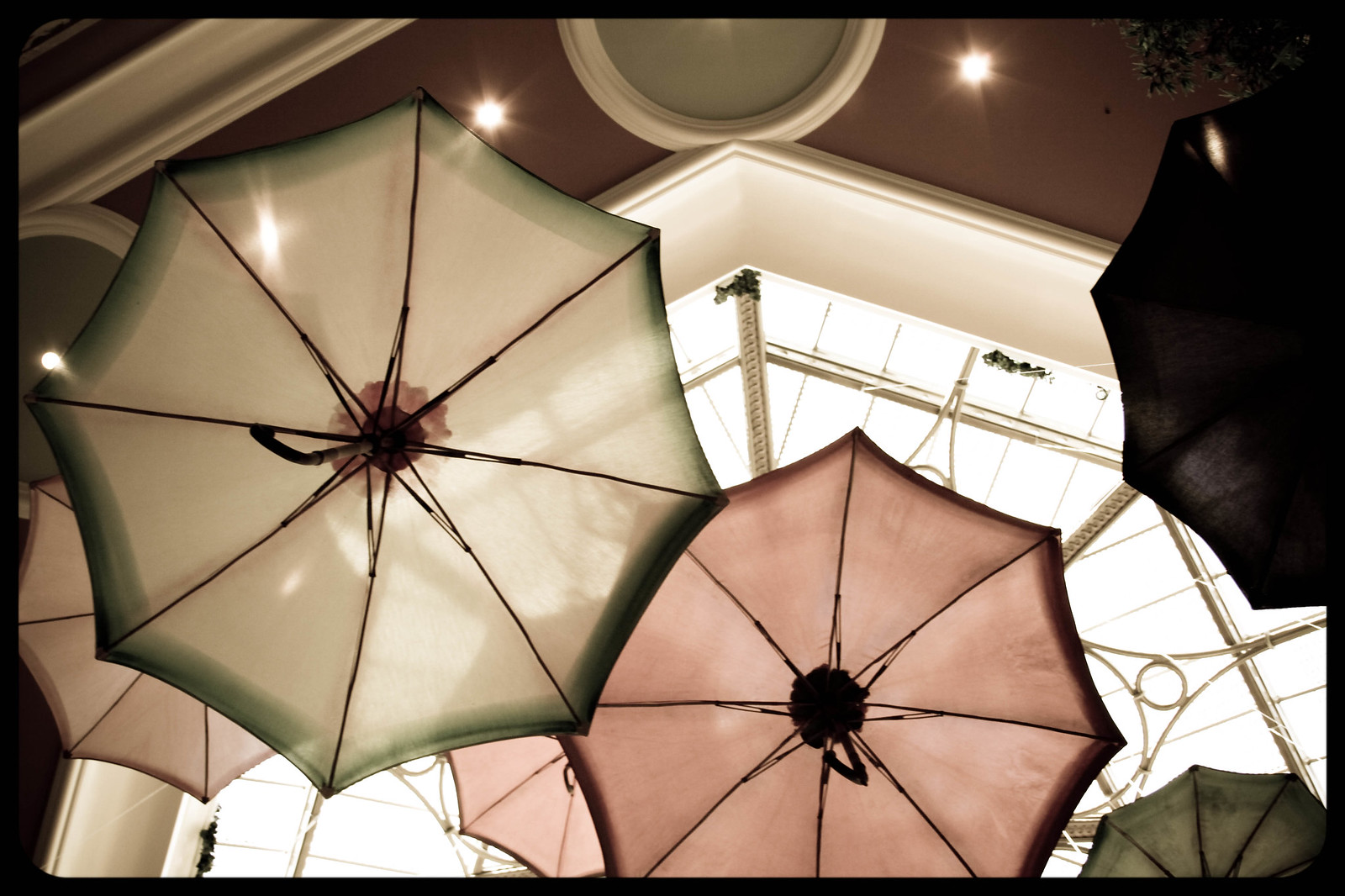This is a detailed indoor color photograph featuring a captivating arrangement of umbrellas suspended from a very tall ceiling. The point of view is from below, looking up at the open umbrellas with their handles facing down towards the photographer. The umbrellas vary in color and design: one on the left is primarily white with a green edge, and another adjacent to it is gray with a greenish-black border. There is a prominent light purple umbrella in the center with a black handle, and similarly colored umbrellas are scattered throughout, including two pink ones in the distance and a green one in the bottom right corner. A black umbrella is positioned on the far right. The ceiling features a massive triangular-shaped window allowing light to stream through. The wall above the window is painted brown, and the roof displays an oval arrangement of small lights and a distinctive circular object in the center with a green interior. The upper left corner of the image reveals a diagonally placed cream-colored skirting board, adding an element of architectural interest to the scene.